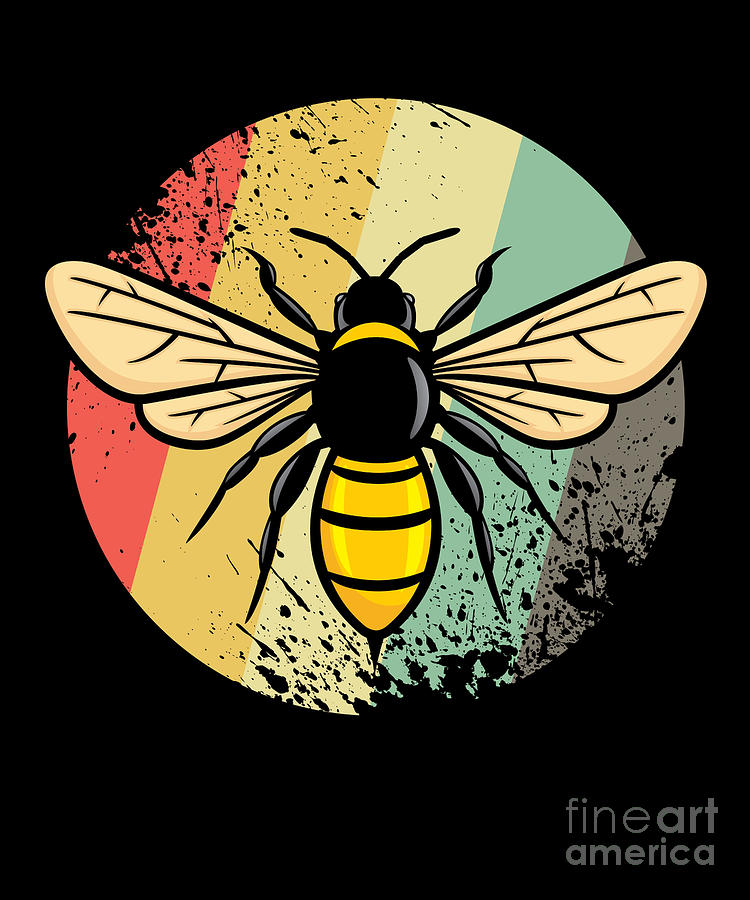The image depicts a digitally illustrated bumblebee, centrally positioned against a stark black background. The bumblebee is yellow with black accents, featuring black stripes and a sharp stinger on the rear. Its head is adorned with white eyes, black antennae, and it maintains a three-dimensional perspective. It has six legs, two positioned at the front and four at the back, with conspicuously detailed wings on each side.

Behind the bee is a large, striking circle with thick, painterly stripes transitioning from pale salmon to pale yellow, cream, light blue, and gray, extending left to right. The circle exhibits black splatters at the top left and bottom right, adding texture and depth to the design.

In the bottom right corner of the image, the text "Fine Art America" appears in subtle gray lettering, further amplifying the image's artisanal quality on what could be described as a tall, rectangular canvas. The entire backdrop remains uniformly black, emphasizing the vivid details and colors of the bumblebee and the striped circle it rests upon.